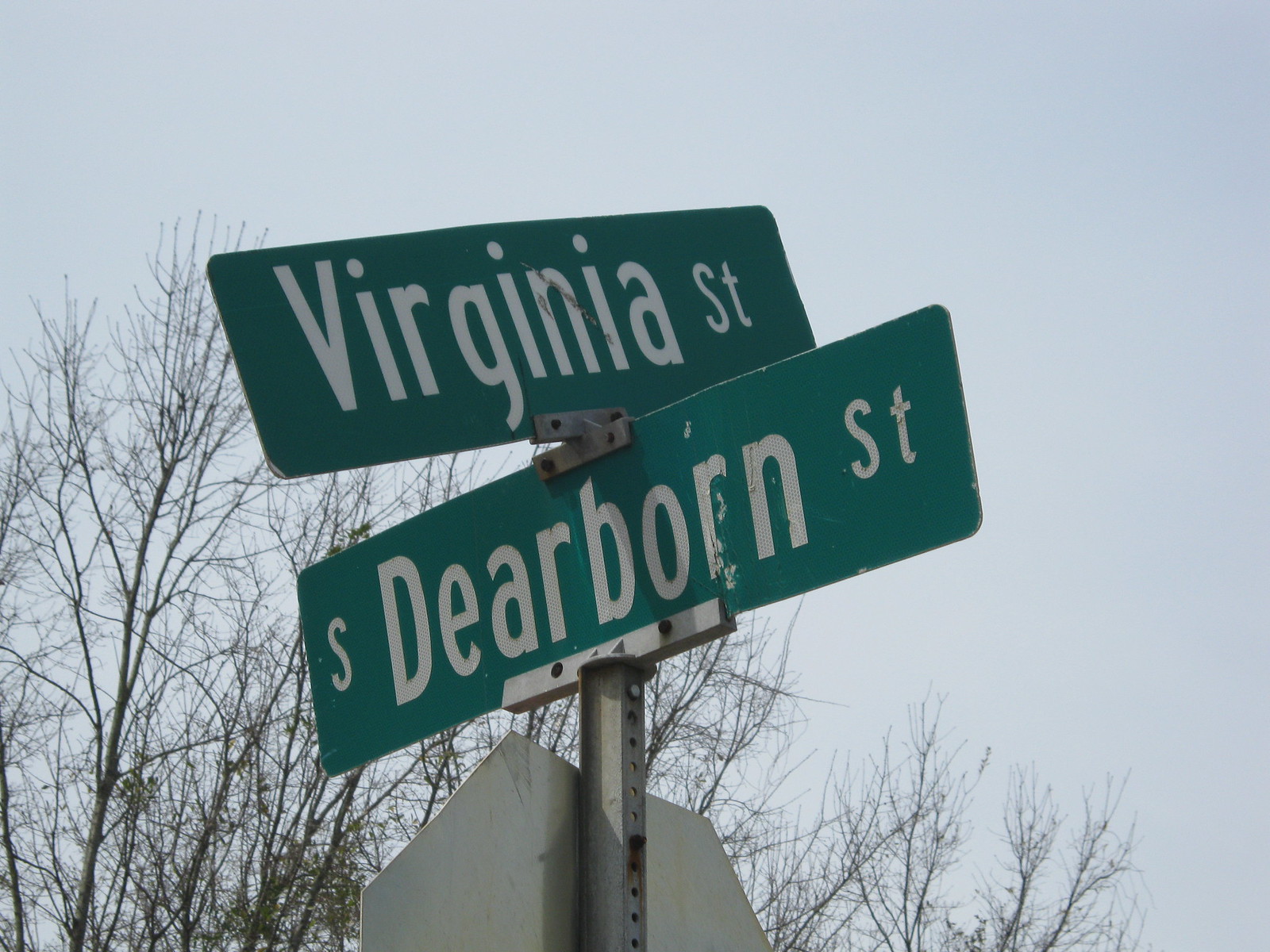This photograph captures a gloomy, overcast day, adding a somber tone to the image of two street signs perched atop a metal post for a stop sign. You can see the hexagonal back of the stop sign, which is facing away from the photographer. The street signs are aligned perpendicularly to each other, with "Virginia Street" on the upper green sign, written in white text, and "S. Dearborn Street" below it, sharing the same color scheme. The signs are mounted on a bracket that holds them in place, though both show signs of wear and tear, including some visible slash marks. The pole appears bent, suggesting it could use straightening. The background is filled with leafless deciduous trees against a gray and cloudy sky, indicative of a cold, possibly wintry day. The overall perspective suggests the photo was taken from a viewpoint looking up at the signs, emphasizing their height and the dreariness of the surrounding environment.